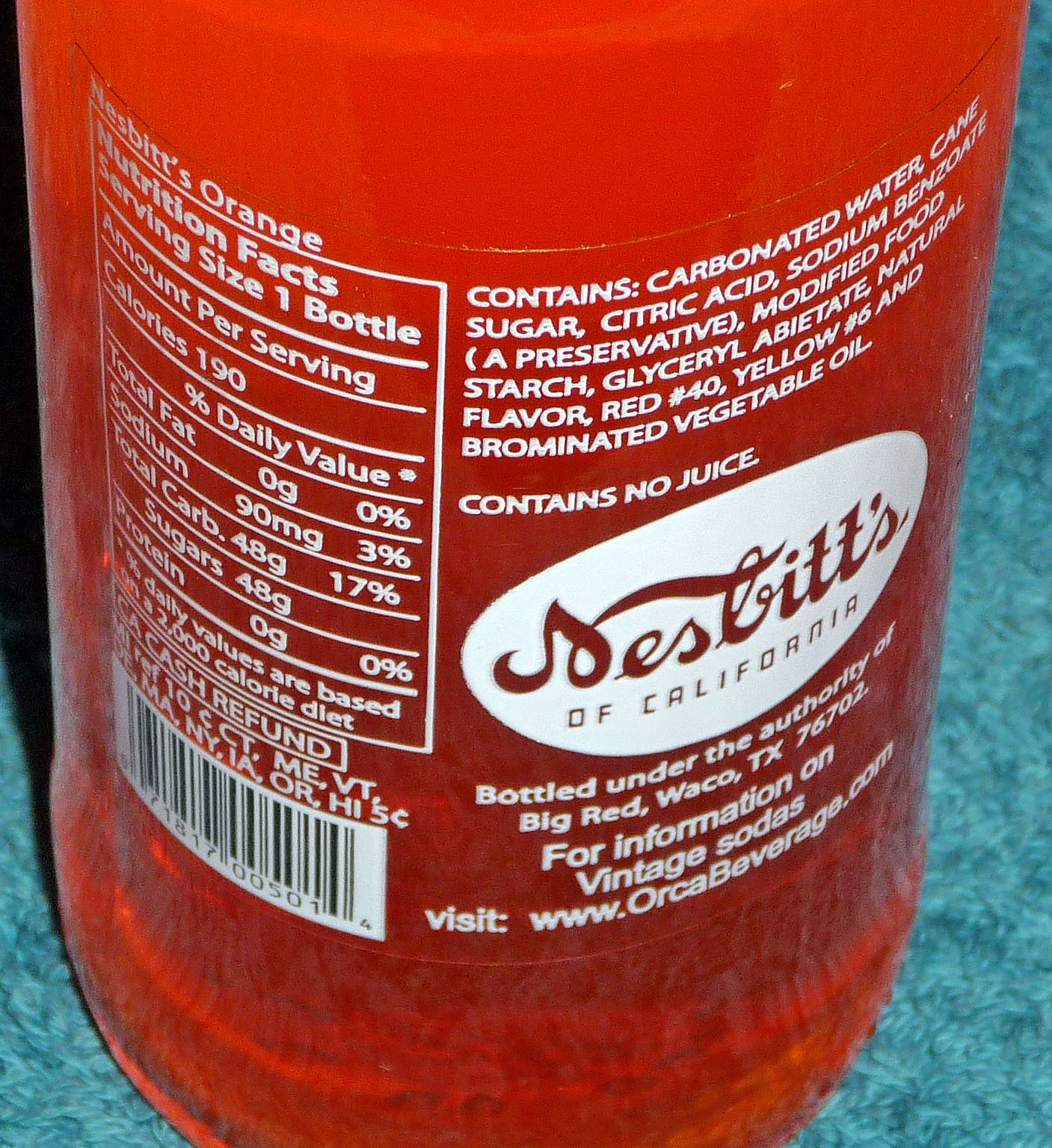The image is a tightly cropped, close-up photo of the backside of a glass drink bottle labeled as Nesbitt's Orange. The bottle showcases the retro logo "Nesbitt's of California," which is depicted in a cursive-like font. The beverage inside appears to be a vibrant red-orange color, and the bottle is placed on a turquoise carpet. Detailed nutritional information is visible on the label, indicating that a serving size is one bottle which contains 190 calories. The ingredients list includes carbonated water, cane sugar, citric acid, sodium benzoate (a preservative), modified food starch, glycerol, natural flavor, Red 40, Yellow 6, and brominated vegetable oil, with a note specifying that it contains no juice. It also mentions that the product is bottled under the authority of Big Red in Waco, Texas, and provides a website for more information on vintage sodas, www.orcabeverage.com. Additionally, a barcode is present on the label.